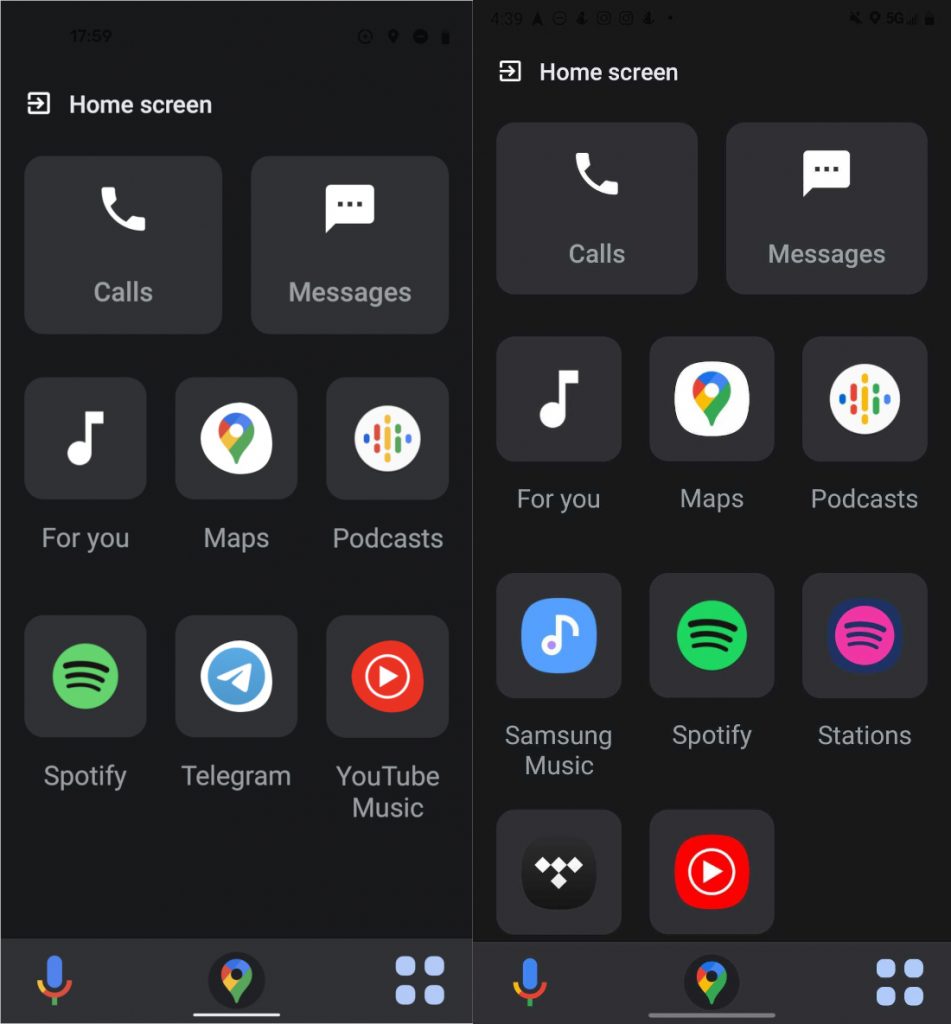**Detailed Descriptive Caption:**

This image showcases a vibrant home screen display with a sleek, black background adorned with predominantly white text. At the very top of the screen, the time is displayed in a clear font, reading "17:59." Below the time, a series of app icons are arranged neatly, each distinctive in color and design, presenting an organized and user-friendly interface typical of a modern smartphone.

The home screen is labelled "Home Screen" and features a variety of apps, each represented by its unique icon. These include: 

- **Calls** - Standard phone icon
- **Messages** - Text bubble icon
- **For You** - Personalized suggestions icon
- **Maps** - Navigation icon
- **Podcasts** - Microphone icon
- **Spotify** - Green circle with black sound waves icon
- **Telegram** - Paper plane icon
- **YouTube Music** - Red play button inside a circular shape

Additionally, at the bottom center of the screen, there are two colorful icons: a microphone and a location pin, both designed in a palette of blue, yellow, red, and green. Adjacent to these are four small blue dots, likely indicating a navigation feature or other interactive elements.

On the other side of the home screen, another array of apps is visible, echoing the primary screen's layout with slight variations in application options. This alternate screen includes:

- **Calls** - Phone icon
- **Messages** - Text bubble icon
- **For You** - Personalized suggestions icon
- **Maps** - Navigation icon
- **Podcasts** - Microphone icon
- **Samsung Music** - Blue music note icon
- **Spotify** - Familiar green and black logo
- **Stations** - Purple radio station icon

In addition to the mentioned icons, there are a couple of notable logos: a black logo and a red logo featuring a play button at its center, enhancing the multimedia capabilities of the device.

Overall, this home screen captures a detailed, colorful representation of a smartphone’s interface, emphasizing a well-organized digital experience with a variety of applications for communication, navigation, music, and entertainment, all set against a minimalistic black backdrop.